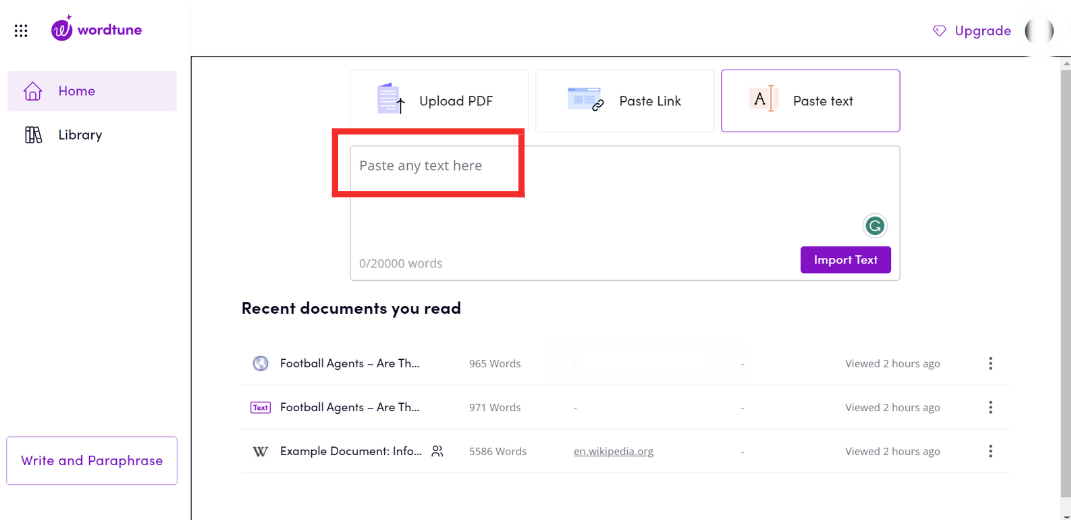The image showcases a detailed interface of the WordChair application. In the top left corner, the WordChair logo is prominently displayed. Below the logo, menu options include 'Home' and 'Library.' The home page features sections for your pets and various functionalities indicated by text commands—'Upload PDF,' 'Paste link,' 'Paste text,' and 'Upgrade.' 

A specific instruction, "Paste any text here," highlighted in red, directs users to input their text. At the bottom left corner, options 'Write' and 'Paraphrase' are clearly available. A designated text field allows for input up to a maximum of 20,000 words, currently sitting at 0 words. Next to this input field, a purple button labeled 'Import Text' is visible.

On the right side of the interface, there are recent documents listed with brief details: "Football Agents," consisting of 965 words, viewed 2 hours ago, another document titled "Football Agents" with 971 words, also viewed 2 hours ago, and "Example Documents Info," with 5,586 words, viewed 2 hours ago. Additional content from the webpage 'an.wikipedia.org' is noted, viewed 2 hours ago.

The entire image is enveloped in a color scheme dominated by purple, red, white, and black, creating a visually structured and organized layout for the user interface.